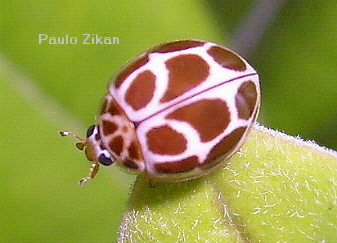This is an extremely detailed close-up photograph of a unique ladybug perched on the very tip of a thick, fuzzy leaf. The ladybug, distinct from the typical red and black variety, displays a striking pattern where its carapace is predominantly white with brown markings, resembling a cow's pattern. The leaf itself is light green with a central seam and light brown accents, covered in fine white hairs, giving it a fuzzy appearance. The background is softly blurred into shades of green, creating a bokeh effect that accentuates the main focus of the image. Curiously, near the upper left of the photo, the name "Paulo Zeikan" is subtly inscribed, adding an additional layer of interest to the composition.